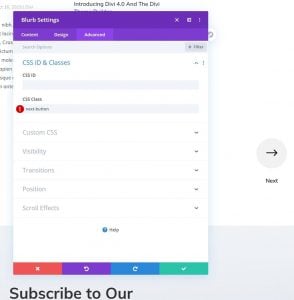The screenshot captures the settings page of a website characterized by a predominantly white interface with a modal window occupying most of the screen. A prominent purple bar stretches horizontally across the top, displaying "Blurb Settings" in white text on the left side. To the far right of this bar, there are three buttons: an 'X' button for closing the pop-up, a square button, and a button with 30 dots, each serving its own function.

Directly beneath the "Blurb Settings" header, the interface features three tabs for navigation. Following these tabs, the options labeled CSS, ID, and Classes offer further customization. Within the main section of the settings page, there are six expandable buttons or sections, allowing for a more detailed configuration.

At the bottom of the menu, a series of buttons corresponding to different actions are present: a red 'X' button for canceling changes, a purple 'Back' button, a blue 'Forward' button, and a green 'Confirm' or 'Check' button for saving changes.